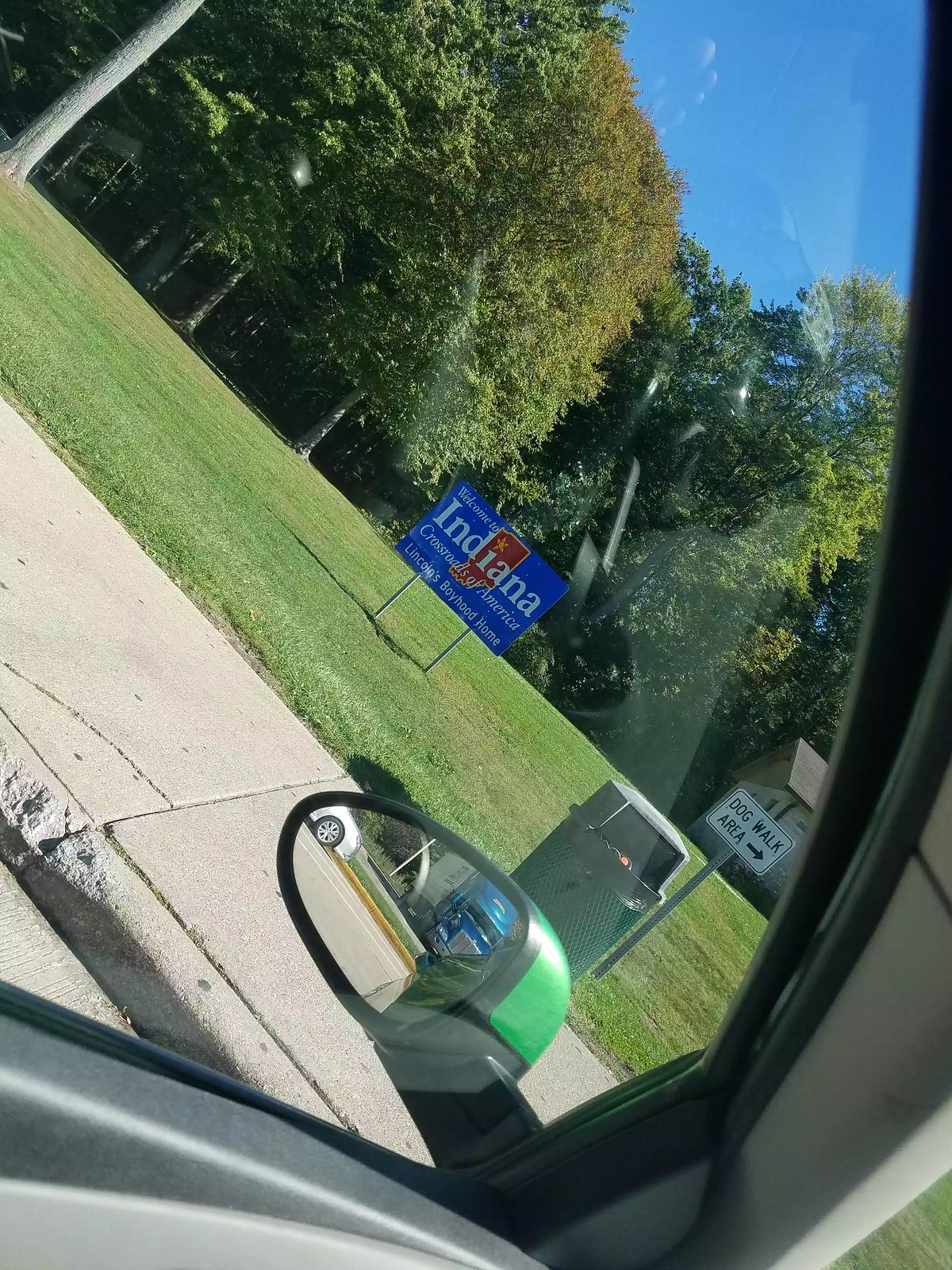Captured through the angled driver's side window of a car, this image prominently features a "Welcome to Indiana" sign situated in an open field. The sign, bathed in a bluish hue, showcases the shape of the state of Indiana prominently in the center, with text underneath reading "Lincoln's Boy Hotel." The scene includes a trash can, positioned towards the right side of the image, along with a designated dog walk area indicated by an arrow, enhancing the roadside ambiance. The photograph’s composition draws attention from the upper left to the bottom right, adding a dynamic perspective to the serene environment.